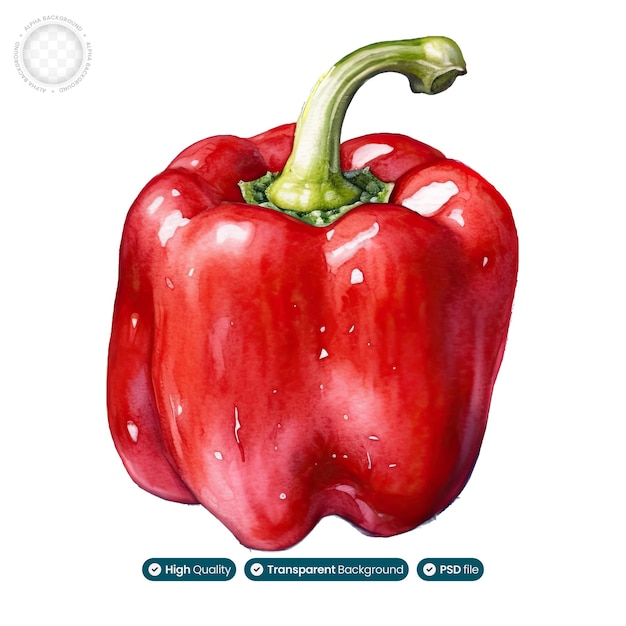This highly detailed illustration depicts a vivid, large red bell pepper with a shiny surface, giving it a realistic and slightly painted appearance. A green stem juts out from the top, curving angularly to the right, indicative of where it broke off during growth. Set against a pristine white background, the image is further characterized by a faded, round gray watermark in the upper left corner. The bottom of the image features three icons with white text on a teal background: "High Quality," "Transparent Background," and "PSD File," all marked with check symbols, denoting the image's attributes.